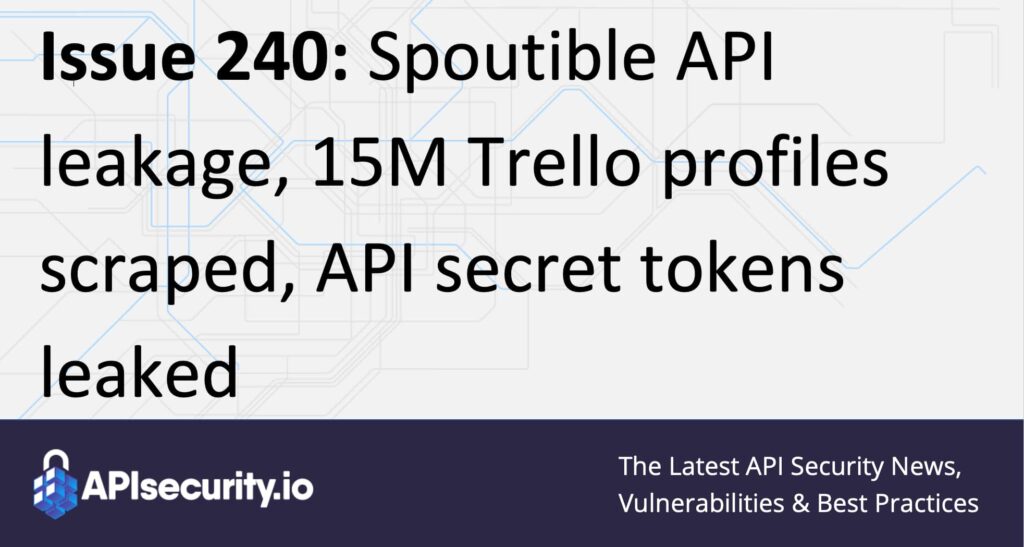This image seems to advertise a security update for the website apisecurity.io. The primary focus is on "Issue 240," which highlights "Spoutable API Leakage," "15M Trello Profiles Scraped," and "API Secret Tokens Leaked." The bolded header text stands out against a faded, pale whitish-blue background adorned with subtle, network-like geometric lines. At the bottom, encased within a navy blue border, the website name "apisecurity.io" is prominently displayed in white text next to a blue and white Rubik's Cube with a lock integrated into the design. To the right of this, it states, "The latest API security news, vulnerabilities, and best practices." The image contains no people or other objects, focusing solely on delivering the critical security information.